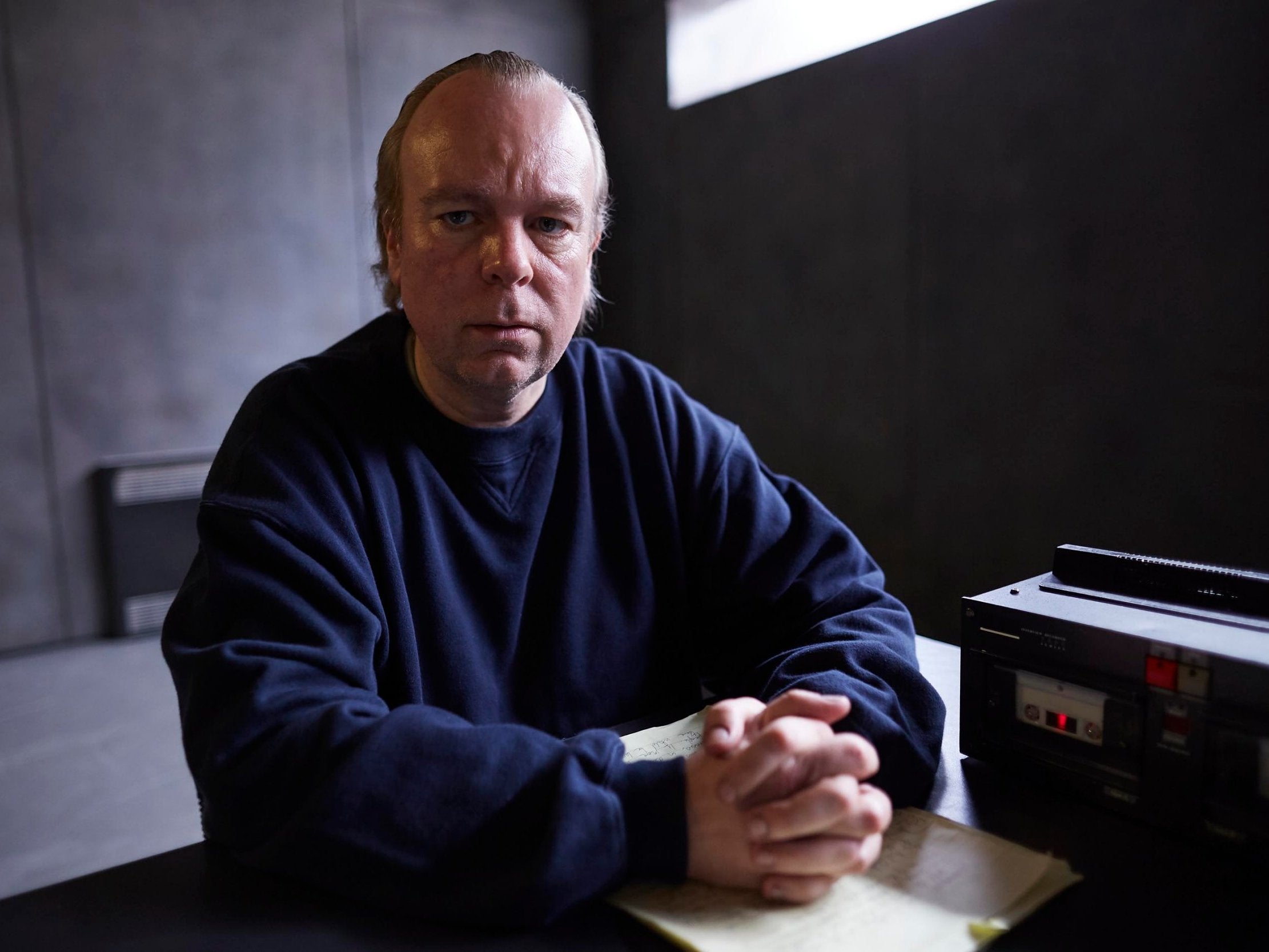In this detailed photograph, an older man, approximately 50 years old, is seated at a dark black wooden table in a dimly lit, grey concrete room with a sliver of white light entering from the upper right. His appearance includes slicked-back blonde hair and a navy blue, long-sleeved sweatshirt. His elbows rest on the edge of the table while his hands are clasped together, interlocking his fingers, and resting on a sheath of rectangular white papers with handwriting on them. The tabletop also holds a boombox with a white tape cassette, positioned next to the man's right arm. A red light and some buttons on the boombox are visible, contributing to the somber and possibly tense atmosphere of the scene. The man gazes upward with a concerned or worried expression. This image appears to be a still from "The Interrogation of Tony Martin," a 2018 Netflix feature, reflecting a style of photographic representational realism.